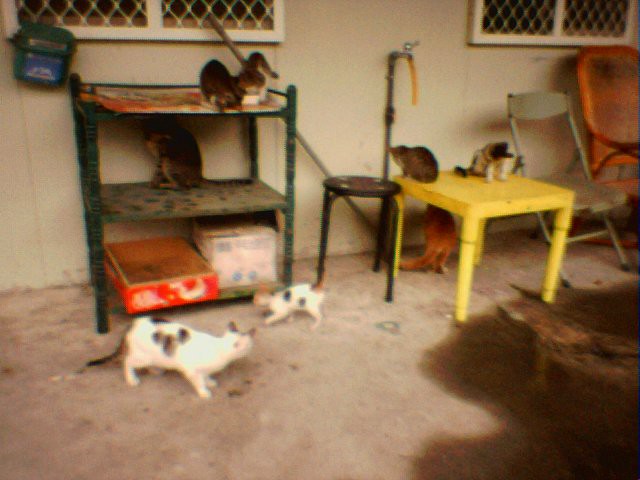This image depicts a cluttered outdoor patio set against a beige house with two large white-framed windows, each covered by metal bars. In front of the first window stands a green, three-shelf wooden unit adorned with 70s-style floral wallpaper. The top shelf houses two small kittens, one calico and one dark black and gray. Below them on the middle shelf sits a gray and black tabby cat, while the bottom shelf holds a red box with white markings and a white cube-shaped box with blue accents. Next to this shelf, a small round black stool sits beside a bright yellow four-legged table. On the table rests two cats; one is black and white while the other is a light brown tabby. Underneath the table lies an orange cat. Adjacent to these furnishings is a metal folding chair in off-white and an orange wicker mat. In front of the shelf, two more cats are visible: one fully grown and the other a kitten, both white with black spots and black tails. The concrete ground, dirty and cluttered, extends throughout the patio, partially obstructed by a white wire and a short length of yellow garden hose hanging from a nearby spigot. Overall, the image features a total of seven cats in various positions both on and around the furniture in this outdoor setting.